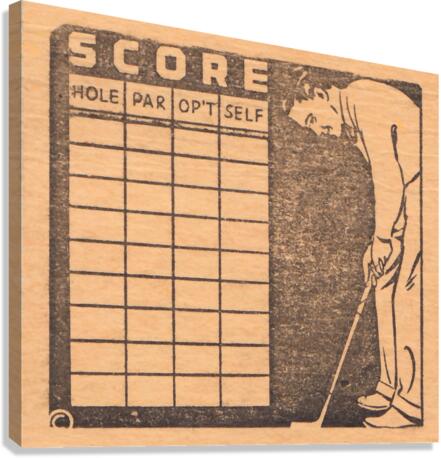This is an image of a scorecard for golf, designed to look like a light wooden plaque with a superficial three-dimensional effect and light gray drop shadow. The scorecard is printed with a black and white graphic that gives the illusion of faded black ink on the wooden surface. At the top left of the card, the word "Score" is prominently displayed. Below this, there is a detailed table with four columns labeled "Hole," "Par," "OPT," and "Self," each containing nine rows for scoring purposes.

On the right side of the scorecard, there's a black and white illustration of a golfer, reminiscent of 1950s attire. The golfer is bent over, holding a putter between his legs, appearing poised to take a putt. The background of the entire image is white, emphasizing the vintage aesthetic of the scorecard, which melds the charm of an old scoreboard with the practicality of a contemporary graphic design.